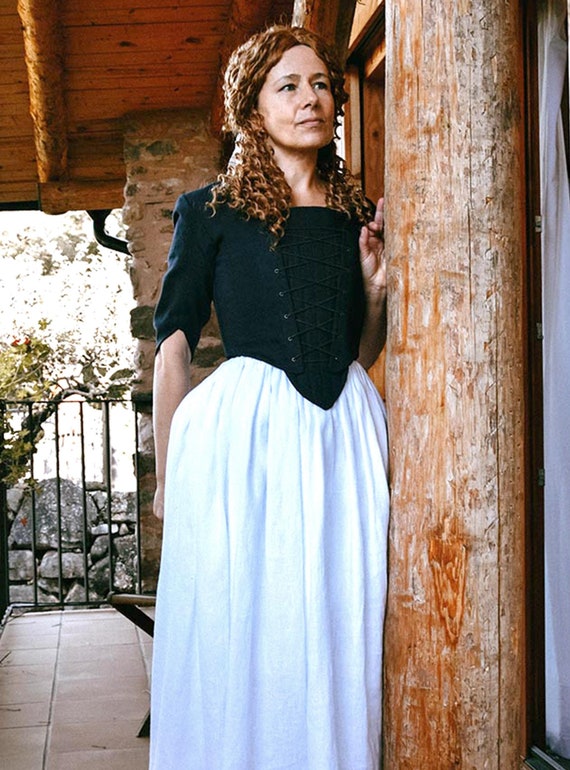This image depicts a white woman with auburn, tightly coiled shoulder-length hair, dressed in period clothing reminiscent of the 1700s or 1800s. She is wearing a fitted dark green bodice with buttons and puffed elbow-length sleeves, which tapers to a peak in front, paired with a gathered, formal white skirt. The outfit bears similarities to garments seen in "Little House on the Prairie." The woman stands on a red-tiled stone patio, leaning against a large, rustic wooden pillar of a log cabin. Behind her is a black cast iron fence and stonework. She gazes intently into the distance, with her hand resting on the column and the other slightly behind her back. A wooden roof overhangs from the left, adding to the rustic setting of the scene.